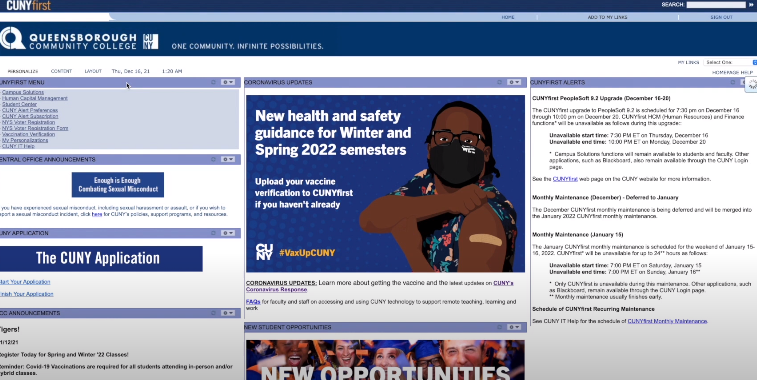Screenshot of the CUNYfirst webpage, displaying the portal for CUNY’s Queensborough Community College with the tagline "CUNY: One community, infinite possibilities." The screenshot captures the date and time: Thursday, December 16, 2021, at 1:20 AM. Several sections are visible, including:

1. **Navigation Menu**: 
   - "My First Menu"
   - "Central Office Announcements"
   - "My Applications"
   - "Announcements"
  
2. **Coronavirus Updates Section**: 
   - Prominent animated icon highlighting new health and safety guidance for the Winter and Spring 2022 semesters.
   - Encouragement to upload vaccine verification to CUNYfirst with the hashtag #VaxUpCUNY.
   - Image of a black woman wearing a black mask and glasses, dressed in a floral attire, displaying her band-aid after receiving the vaccine.
   - Call to action: "Learn more about the vaccine and the latest updates in CUNY’s coronavirus response."

3. **FAQs for Faculty and Staff**: 
   - Guides on assessing and using CUNY technology to support educational activities.

4. **CUNYfirst Alerts Section**: 
   - A category dedicated to urgent updates and alerts for users of the CUNYfirst system.